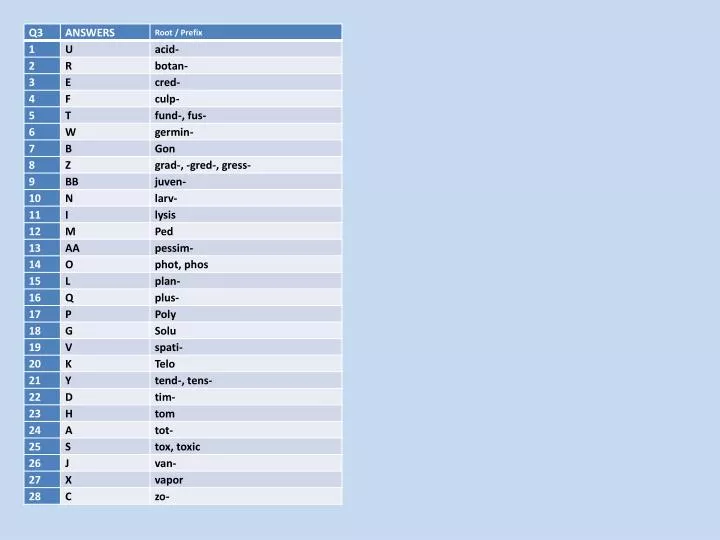This is a detailed photo depicting a wide vertical panel on a very large light blue square, positioned to the far left. The panel is divided into three distinct columns. The first column, labeled "Q3" at the top left, lists 28 numerical entries vertically. Directly to the right, the second column is labeled "Answers," containing a corresponding vertical list of letters. The third column on the far right is labeled "Root/Prefix," which provides a vertical list of root words and prefixes that align with the respective numbers and letters in the other two columns. For example, the first entry under "Q3" is paired with an answer "U" in the "Answers" column, and the root prefix "acid" in the "Root/Prefix" column. The second entry under "Q3" matches with "R" in the "Answers" column, and the root prefix "botan" in the "Root/Prefix" column. The organized layout ensures clear and easy reference to questions, their answers, and corresponding root words or prefixes.